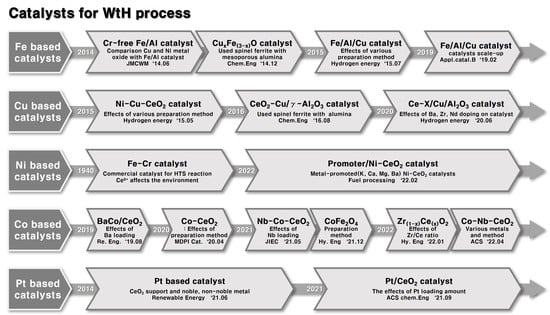The image is a detailed scientific diagram titled "Catalyst for WTH Process." It consists of a flowchart with a white background, with the primary elements outlined in dark gray and labeled in white and black text. The chart depicts a horizontal progression of various metal-based catalysts used in a specific chemical process, denoted as "WTH."

Starting at the top left, the metals listed are:

1. **Fe-based catalysts (Iron)**
2. **Cu-based catalysts (Copper)**
3. **Ni-based catalysts (Nickel)**
4. **CO-based catalysts (Cobalt)**
5. **Pt-based catalysts (Platinum)**

Each of these categories is connected by thick, arrow-shaped boxes outlined in dark gray, pointing rightward. Within these boxes are detailed compositions and specific types of catalysts derived from each base metal. The chart also includes significant years, such as 2014, 2015, 1940, 2019, 2014 again, and more, which likely indicate the years when these catalysts were used or introduced.

Overall, the flowchart illustrates a timeline and comparison of different catalysts, showing the dates and specific variations or formulas of each catalyst type in a structured, arrow-based format. This detailed visual representation helps in understanding the evolution and application of metal-based catalysts in the WTH process.